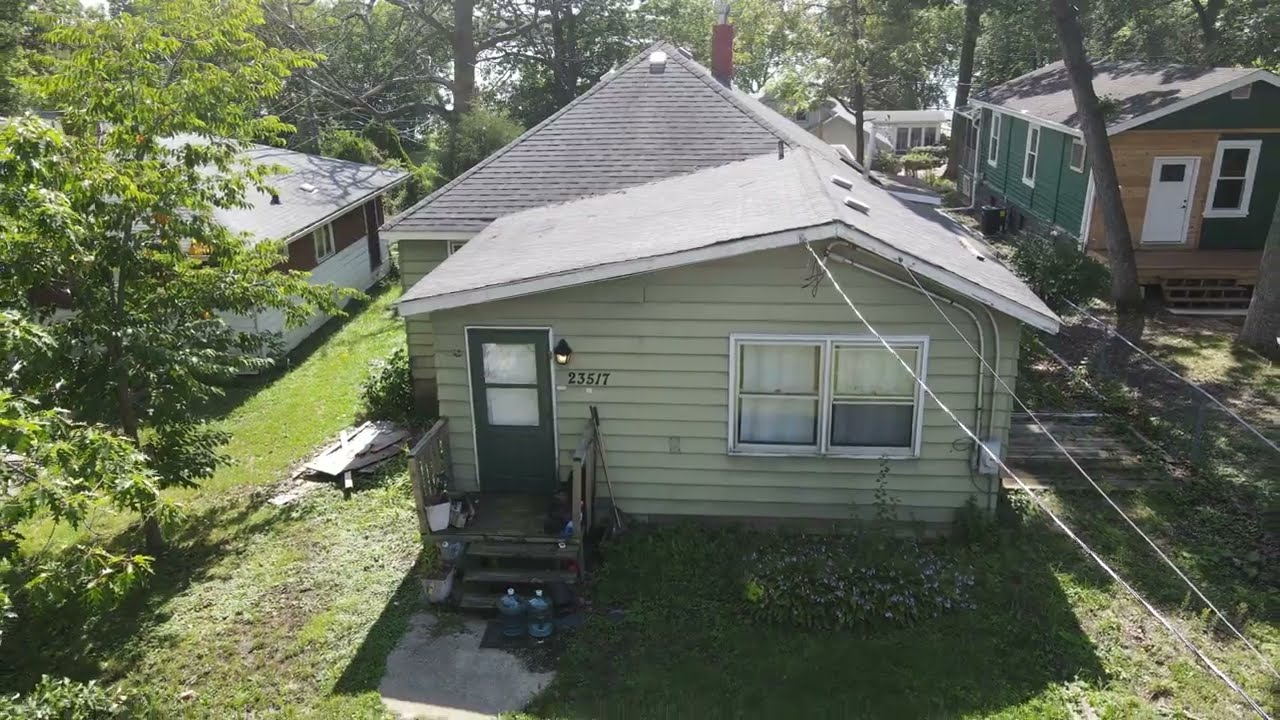The aerial photograph captures a detailed overhead view of a neighborhood dominated by a single-story, older-style house with light green siding and a dark green front door positioned on its left side. The house, which occupies the center of the image, is bathed in bright sunlight, slightly fading the roof's appearance and revealing a chimney towards the back. The front yard features a grass lawn, flanked by narrow lawns on either side, with approximately 10 feet separating the house from its neighbors. To the immediate left of the house, a tall tree extends up the side of the image, partially concealing a second house sitting on a lower elevation, characterized by white and brown tones. On the right edge of the image, the third house displays dark green siding with a white door and brown wood surrounding it, indicating unfinished painting. The front steps of the central house are adorned with numerous potted plants, while in the foreground, cables run from the right towards the house. The neighborhood hints at an East Coast ambiance, with an evident yet subtle touch of vintage charm and potential construction or renovation undertakings in the vicinity.